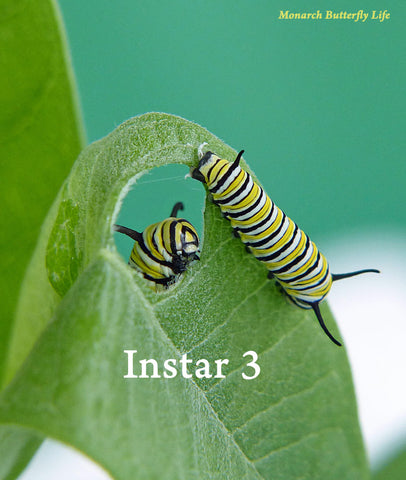This vivid nature photograph, titled "Monarch Butterfly Life," showcases two monarch butterfly caterpillars adorned in striking yellow, white, and black stripes. They are both actively feasting on a bright green leaf, creating noticeable holes as they chew through it. One caterpillar is positioned on the backside of the leaf, having already made a large hole, while the other begins to eat on the front side, its antennas distinctly visible. The leaf, slightly bent, is complemented by another upright leaf in the softer, mint-green background with white accents. The leaf also bears white text that reads "In Star 3," indicating the stage of the caterpillars' development. The overall composition blends the vibrant green foliage with the serene blue and white hues of the backdrop.